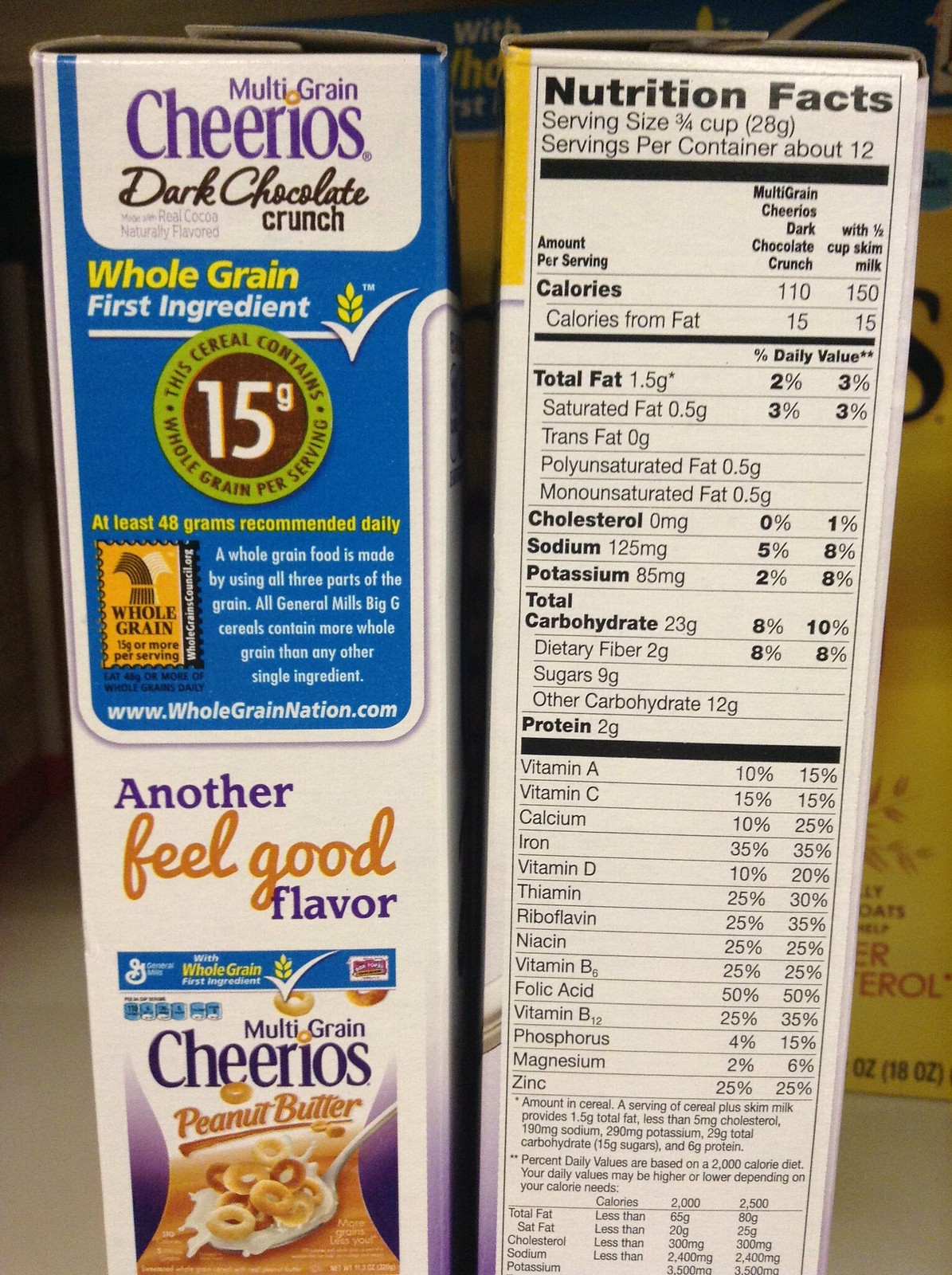The image showcases the sides of two cereal boxes in great detail. The first box prominently displays the label "Multi-Grain Cheerios" with the specific variant being "Dark Chocolate Crunch." It highlights the health benefits, stating that "Whole Grain" is the first ingredient and each serving contains 15 grams of whole grains, noting that the recommended daily intake is at least 48 grams. Additionally, the box promotes another variety underneath, "Multi-Grain Cheerios Peanut Butter," as "another feel-good flavor."

The side of the second cereal box presents nutritional information for a different cereal. It specifies the serving size as 3/4 cup, with about 12 servings per container. The detailed nutrition facts reveal that each serving contains 110 calories, which increases to 150 calories when combined with skim milk. It provides extensive information on calorie content, fat percentages, and an array of vitamins and other typical cereal ingredients.